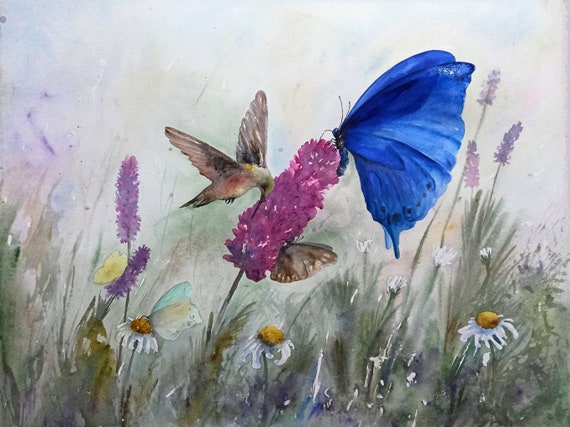This watercolor painting captures a serene field of wildflowers beneath a subtly dreary sky. The rectangular canvas, slightly wider than it is tall, showcases a variety of muted green hues—ranging from muddy greenish-gray to olive tones on both the left and right sides—representing the untamed grass. Interspersed throughout this earthy expanse are numerous white flowers with yellow centers, adding a soft contrast to the greenery. Dominating the center of the scene is a large, cone-shaped lavender flower that draws immediate attention. 

To the left of this striking purple bloom, a brownish hummingbird with a green head hovers delicately, poised in mid-air. On top of the flower, a vibrant blue butterfly is perched, adding a splash of color and intricacy to the composition. Lower down, near the base of the flower, another smaller butterfly, brown in color, can be seen. The upper half of the painting transitions to a sky rendered in shades of white and light blue, suggesting either an overcast day or the calm before a storm, enhancing the tranquil yet somber atmosphere of the piece.